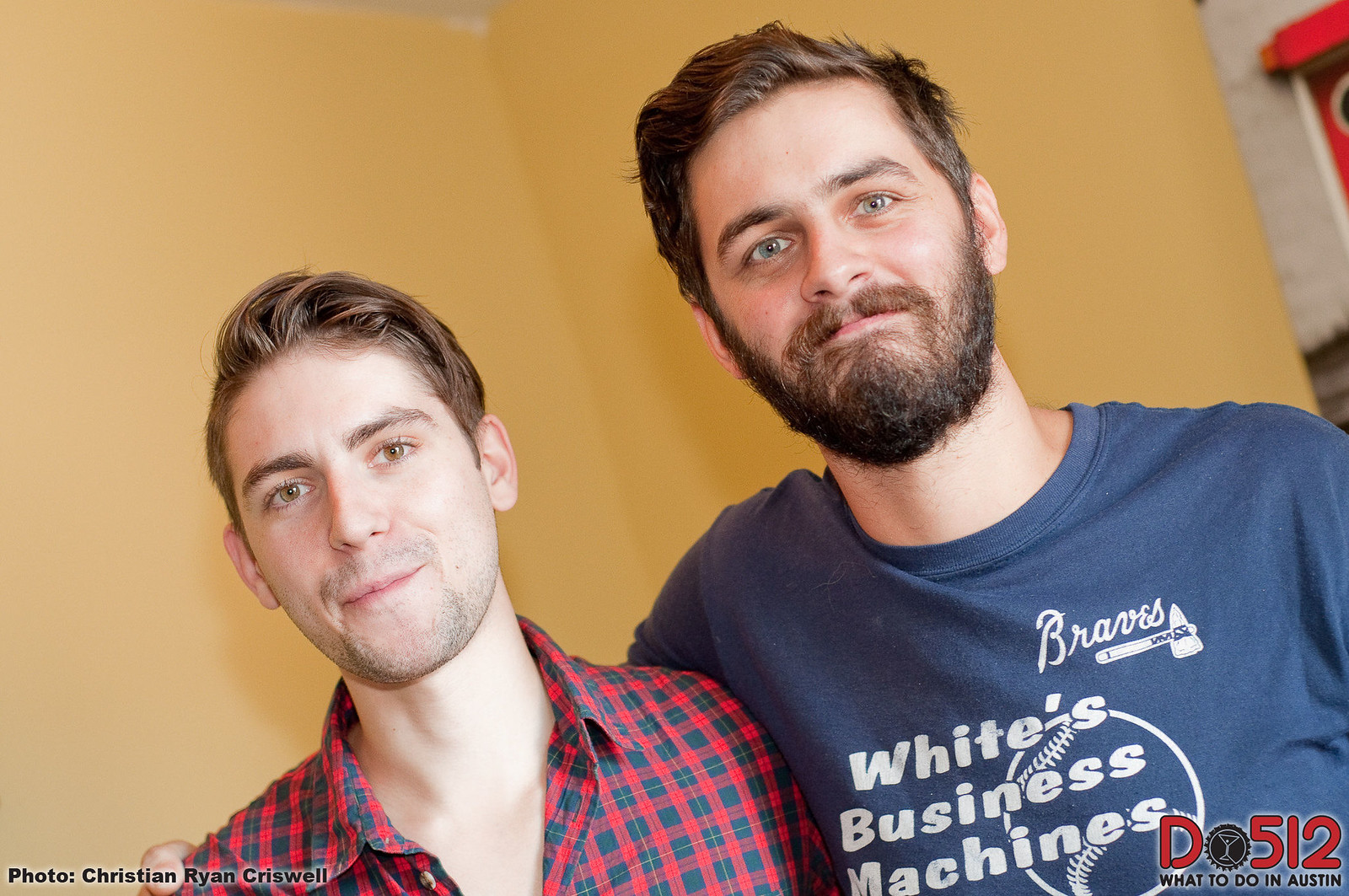This photo showcases two young Caucasian men posing together against a yellow wall, their image captured at a 45-degree diagonal angle, tilting upward to the right. Both men are in their early twenties and have fair complexions. The man on the left, who has dirty blonde hair and light stubble, is wearing a red and blue plaid shirt. He appears thinner and has a youthful appearance with fresh-looking skin. The man on the right, sporting a full beard and bright green eyes, has brunette hair and is dressed in a dark blue t-shirt featuring a graphic of a baseball and the text "Braves" along with "White's Business Machines." His arm is affectionately draped around his friend's shoulder. In the bottom corner of the photo, a watermark reads "Photo: Christian Ryan Criswell," accompanied by the logo and text "D0512," and the phrase "What to do in Austin." The image captures a casual, commemorative moment between the two friends.